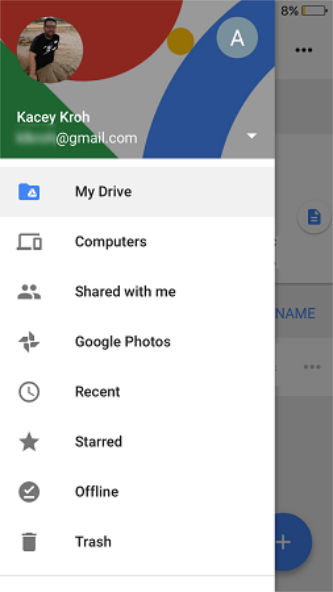Close-up view of a Google profile interface on a computer screen. In the top left corner, there is a profile picture of a man with short black hair, a short beard, and a mustache. He is wearing glasses and a black t-shirt with white designs on the front, paired with sandy-colored cargo pants. The photo appears to be taken in a dark room with a brownish, grassy field visible in the background. 

To the right of the profile picture, there is an 'A' within a gray circle and the name "Casey Kroch," followed by an obscured email address ending in "@gmail.com." Below this, the "My Drive" section is currently selected, highlighted in blue, amidst other gray icons. The visible icons include:

- Computers (depicted as a computer screen and a cell phone screen)
- Shared with Me (represented by two person icons)
- Google Photos (a small fan icon)
- Recent (a clock icon)
- Starred (a star icon)
- Offline (a circle with a tick mark)
- Trash (a trash can icon)